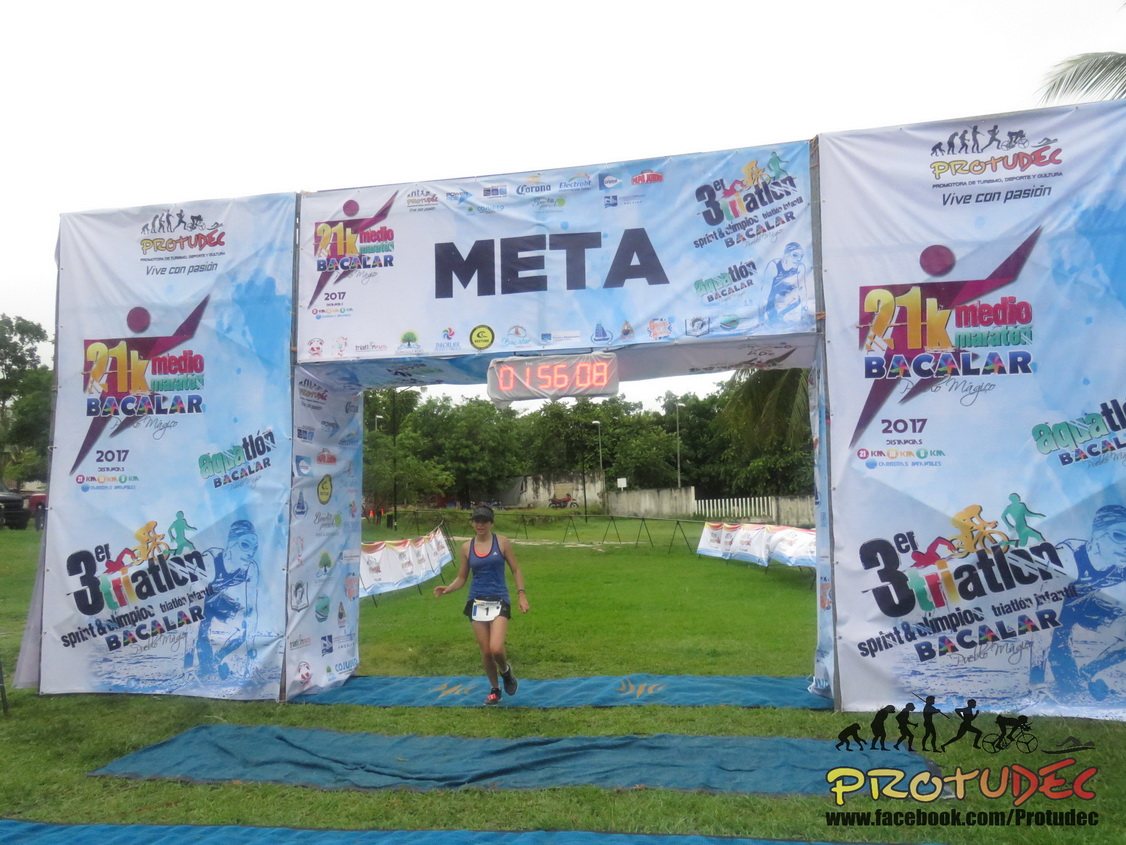In this vibrant image, a woman in athletic gear is captured triumphantly crossing the finish line of the 21k Meta Marathon Beclair 2017, prominently displayed with the text "META 2017" on the arched structure overhead. This finish line arch is adorned in white and blue, featuring various sponsor logos, including Papa John's, and a timing clock showing she completed the marathon in one hour, 56 minutes, and eight seconds. The runner, positioned centrally in the photograph, is outfitted in a blue tank top, black shorts, and a blue hat, with her race number visible around her waist. The ground underneath her features scattered carpets on a grassy surface, and the outdoor race setting is bright and lively with an array of colors such as white, gray, green, dark blue, blue, purple, pink, orange, and yellow. Additionally, the bottom right corner of the image contains a logo and text promoting Pro2Dec's Facebook page.